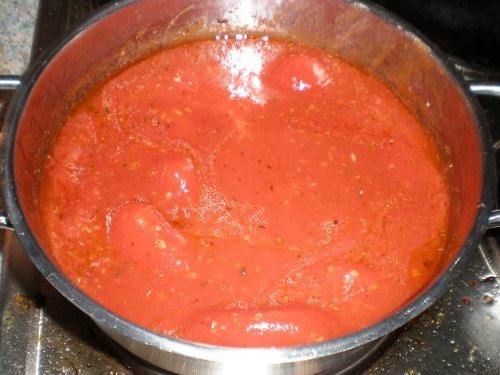The image depicts a close-up, rectangular photograph of a large, stainless steel pot positioned on a stove. Captured from an overhead angle, the photo highlights the pot brimming with a thick, deep red marinara sauce. The sauce has visible herbs and spices mixed throughout and appears to be close to boiling, with some bubbling discernible near the surface. The pot features silver handles on both the left and right sides, although parts of the handles are cut off due to the close framing of the shot. Surrounding the pot, the stove area appears quite dirty, with noticeable food particles, grease, and splatter. The backdrop includes a mostly black countertop and possibly some grid-like structures, indicating the indoor setting might be a kitchen or a restaurant. The primary colors in the image are black, white, red, and silver.